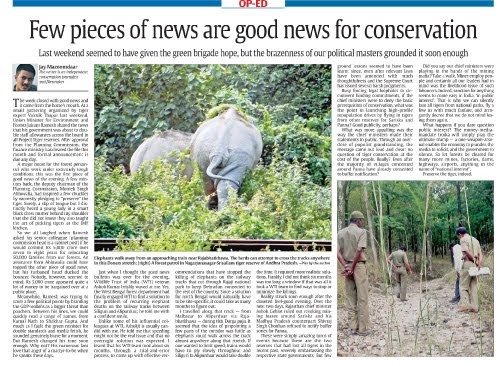This image is a scan of a newspaper article with a white background at the top. The page features a medium blue bar running across its width, which is interrupted in the center by a white rectangle. Inside this white rectangle, there's bold red text in all caps reading "OP.ED," and just below it is a light gray rectangle. At the top of the article's body, there's black text stating, "Few pieces of good news are good news for conservation." Centered beneath this is a smaller line of text that reads, "Last weekend seemed to have given the Green Brigade hope, but the brazenness of our political masters grounded it soon enough."

To the left of this text is a square photograph showing a man's face. Adjacent to the right of the photograph is some bolded black text, although it's too blurry to be legible. Below this bold text are three lines of smaller black text, which are also too blurry to read. A thin black line extends from the bottom of the photograph toward the right. Underneath this line is a series of paragraphs in standard newspaper print, but the text is too blurry to read except for the first letter, a large dark gray capital "T."

In the center of the page is another square photograph, this one depicting the rear ends of two elephants walking into a forest. The elephants are surrounded by a sea of green leaves, and at the bottom of the image, there is a horizontal brown beam, possibly resembling a railroad track or a similar structure.